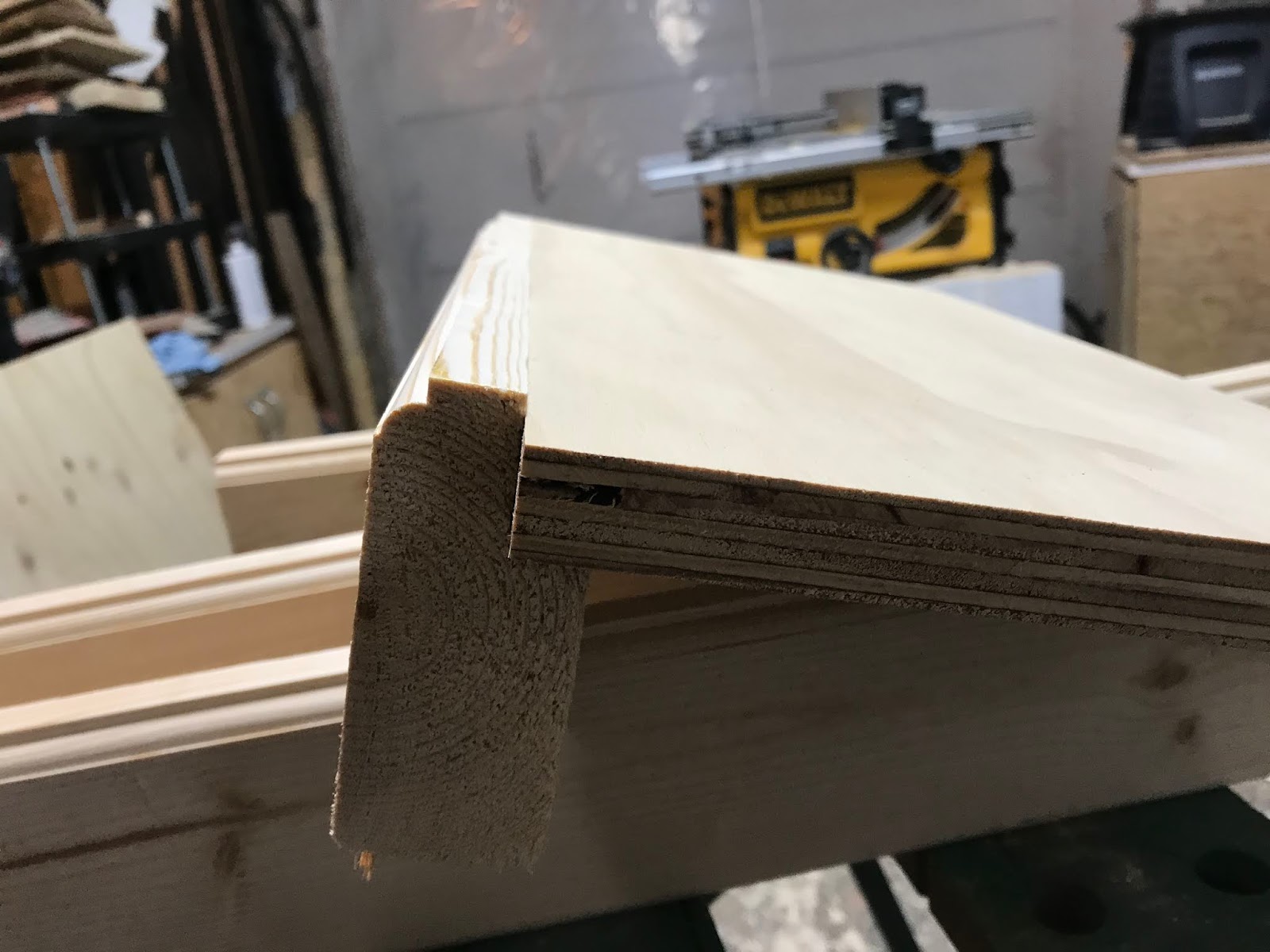In this image, we see a detailed woodworking setup. At the center, there's a sheet of plywood mounted onto a two-by-four. The background features an off-white wall. A DeWalt small table saw is prominently displayed, identifiable by its yellow base, black handle, and silver top and cutting guide. To the right, there's a small plywood table with an indistinct black and gray object on top, possibly a box. The table saw itself appears to be resting on a box, partially obscured by the foreground wood.

Directly in front of us are two-by-fours with beveled edges, giving them a rounded appearance, all in a light wood tone. Further to the left, there's a sheet of plywood showing natural knots and a distinctive grain pattern with light white fibers running vertically. Additionally, a black shelving unit is visible on the left side, positioned atop brown cabinet doors with silver metal handles. This detailed setup showcases an organized workspace with various materials and tools ready for woodworking projects.